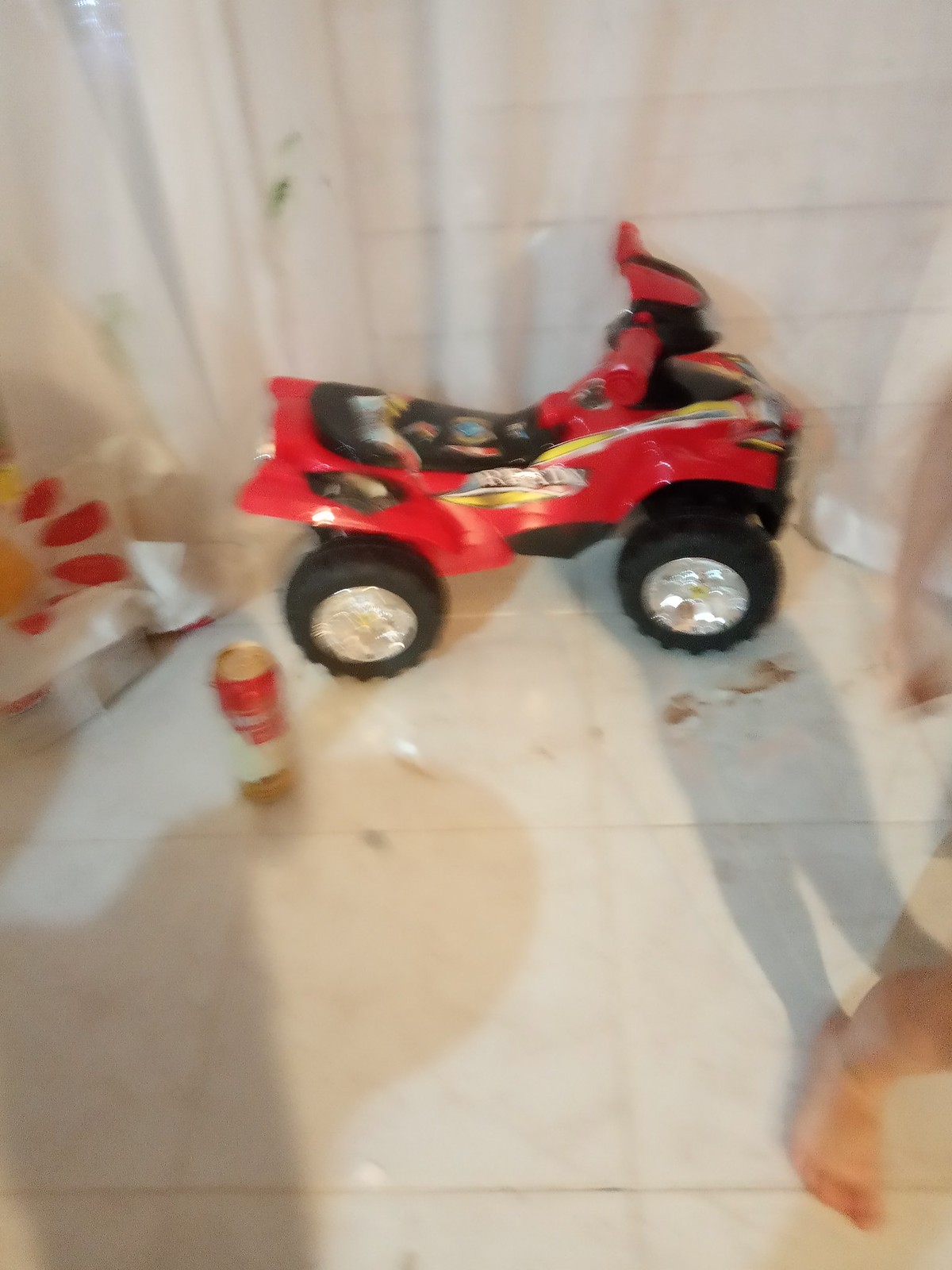This detailed image showcases a child's electric ride-on toy resembling a motorbike, prominently displayed in the center and back center of the photograph. The toy, painted in bright red, features a single seat and is sized appropriately for a toddler. It rests on what appears to be a linoleum floor, suggesting the scene might be set on a porch. The floor has visible tire tracks, indicating some recent play. A white curtain hangs behind the toy, adding a soft backdrop to the scene.

To the right of the motorbike, there is a white bag with distinctive red and yellow petal patterns, reminiscent of a Chick-fil-A bag, possibly holding a pillow or other soft item inside. Additionally, a can is positioned next to the toy, emphasizing the motorbike's small stature. While the mode of propulsion—whether battery-operated or manually powered by the child's feet—is not clear, the overall scene vividly captures a moment from a child's play area, blending everyday household objects with playful elements.